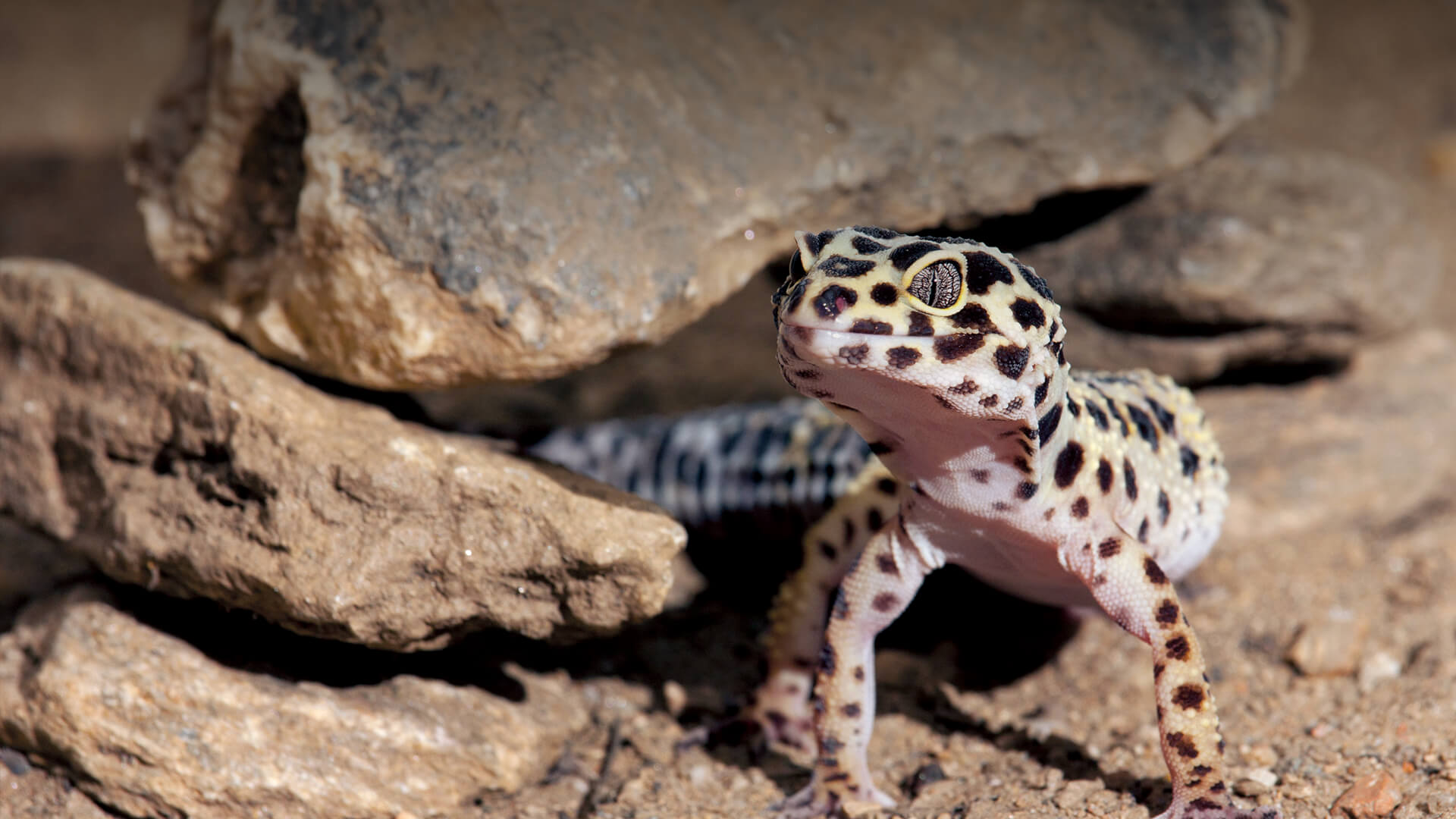In this detailed image, we observe a gecko emerging from an opening at the bottom of a stack of rocks in a desert-like area, with a sandy ground. The gecko's striking appearance features a predominantly creamy white base color, adorned with intricate black spots that are scattered across its body, head, and legs, reminiscent of a leopard or cheetah pattern. Its eyes are dark, raisin-like, and gleaming, adding a contrast to its vivid skin. The tail of the gecko has a striped pattern, combining black and white with touches of the creamy color found on the rest of its body. The rocks surrounding it are grayish-brown, enhancing the natural, rugged terrain. The gecko remains perfectly still, basking in the sunlight, an image that encapsulates the serene and hardy life of desert reptiles.